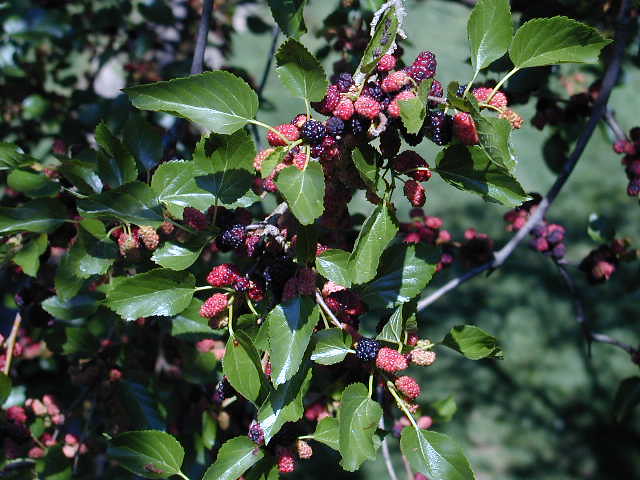The photograph captures a vibrant tree, or possibly a bush, abundant with a mixture of black and red berries. The berries vary in ripeness, with blackberries indicating full maturity and the red ones still in earlier stages, shaded from light maroon to reddish-pink. The branches, primarily a dark gray color, appear robust and healthy, supporting a profusion of green leaves. These leaves are distinctly veined, with lighter, almost tan veins and slightly curled, jagged edges which give them a sharp appearance. Smaller secondary branches can also be seen, though the background blurs into a wash of green, suggesting the presence of grass and potentially another similar berry-laden plant. The photograph exudes a sense of natural, organic growth prevalent in wild environments, contrasting the smaller, naturally-grown berries with the larger varieties often found in grocery stores.